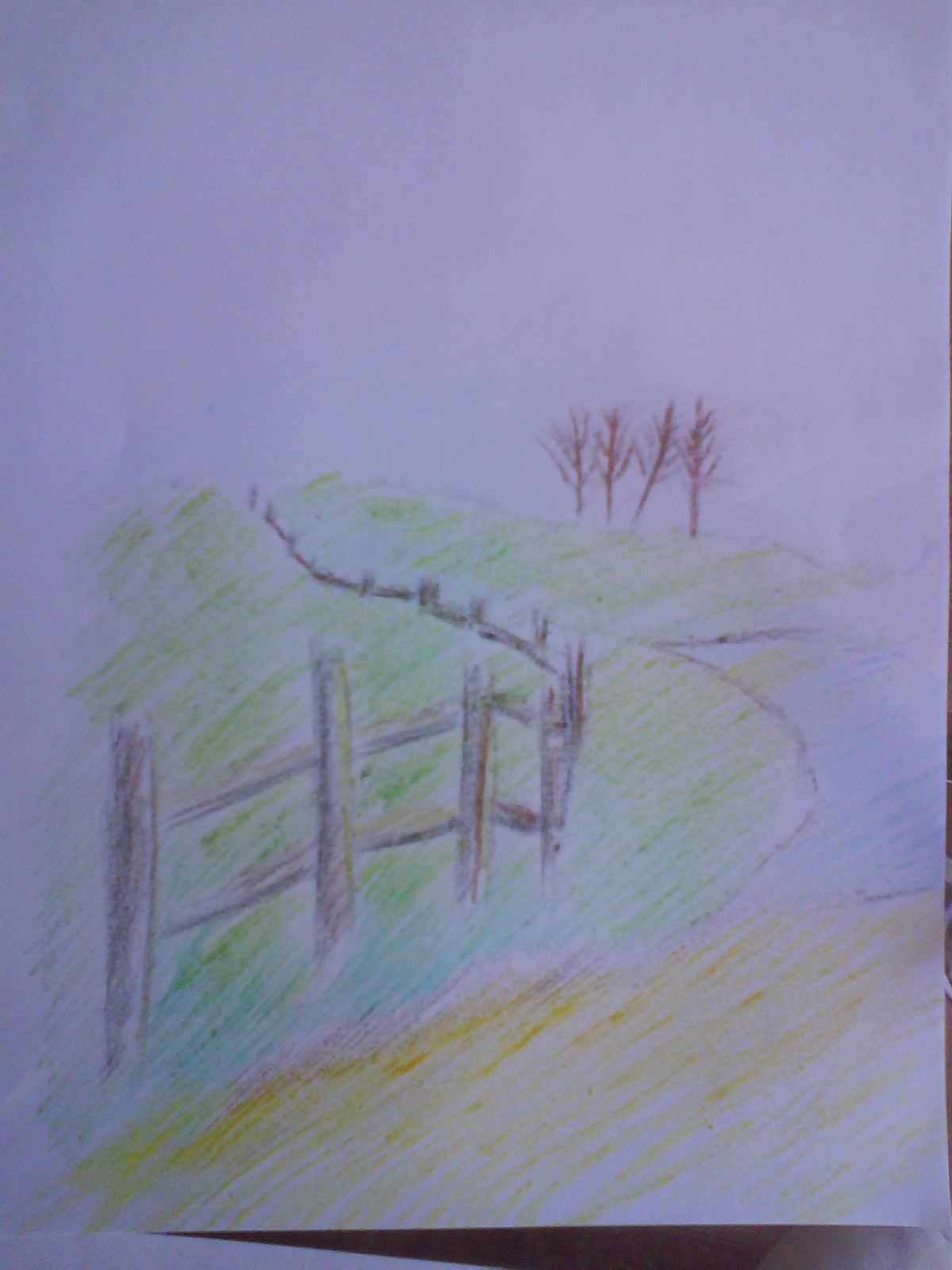This image is a color snapshot of a child's drawing on a white piece of paper, partially tinted in magenta and light blue pastel hues due to low lighting. The drawing, done in crayon and possibly colored pencil, portrays an outdoor countryside scene covering the bottom two-thirds of the paper, leaving the top portion white and unfinished, suggesting a plain sky.

In the foreground, a yellow path or road snakes upward, curving to the right and blending into a blue area that could represent a different part of the road or water. Parallel to this path, a wooden fence with brown posts stretches back into the distance from the middle left side of the paper, creating a sense of depth. The fence is detailed with alternating horizontal and vertical posts, adding structure to the landscape.

Green grass flanks both sides of the path and lines the base of the hills in the background. Among the hills, four bare brown trees stand on the horizon, their branches reaching up without leaves, giving the drawing a simple yet poignant touch.

The colors are applied loosely with diagonal shading in yellow, light blue, purple, green, and brown, adding texture and dynamism to the scene. Despite the lack of detailed coloring and the unfinished sky, the drawing vividly captures the essence of a tranquil countryside view.